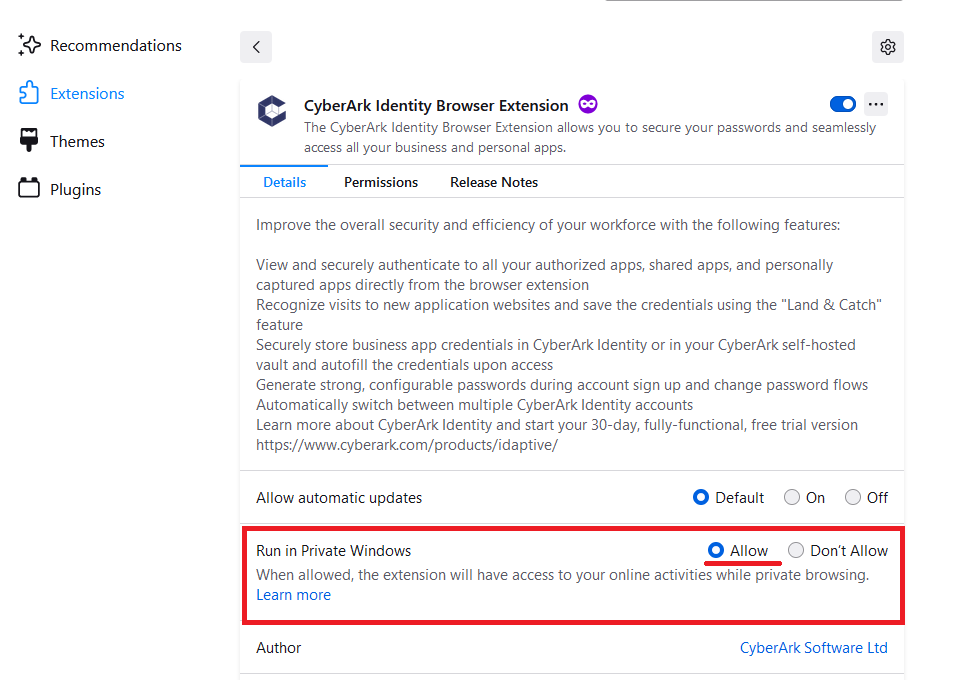A detailed screenshot of a browser interface is shown, highlighting the "Extensions" tab in a list on the left side of the screen. The extensions section is accentuated with a blue border, indicating it is selected. Among the various extensions, the "CyberArk Identity Browser Extension" is prominently featured. The CyberArk logo, which is a stylized 'C' in navy, dark blue, or black, is visible. The extension is described with a brief summary: "The CyberArk Identity Browser Extension allows you to secure your passwords and seamlessly access all your business and personal apps."

Below this description, detailed features of the extension are listed. These features include the ability to securely view all authorized, shared, and personally captured apps directly from the browser extension. It also recognizes visits to new application websites, assists in saving credentials, and automates the creation of logins using handy tools. Additionally, the extension supports the storage of business app credentials and the management of multiple identity accounts simultaneously. Users can also utilize it in private browsing windows. The interface ensures that users can learn comprehensively about the functionalities and benefits of the CyberArk Identity Browser Extension.